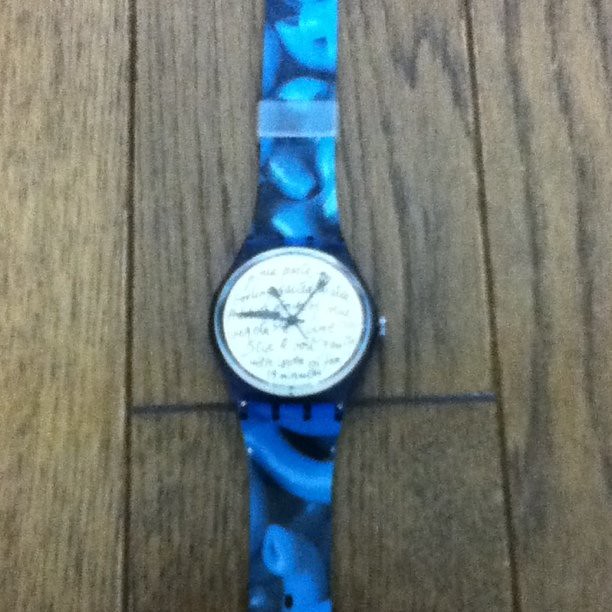On a walnut-colored wooden floor lies an intriguingly designed wristwatch. The watch features a band adorned with a mesmerizing psychedelic blend of light, medium, and dark blue hues. The watch face, although lacking traditional numerical markers, is covered with an array of indistinct scribbles, giving it a mysterious and abstract appearance. The timepiece is equipped with hour, minute, and second hands, and includes a functional stem on its right side for adjustments. The band secures with a clasp mechanism, and is fitted with a sliding loop to manage any excess length, ensuring a neat appearance when worn.